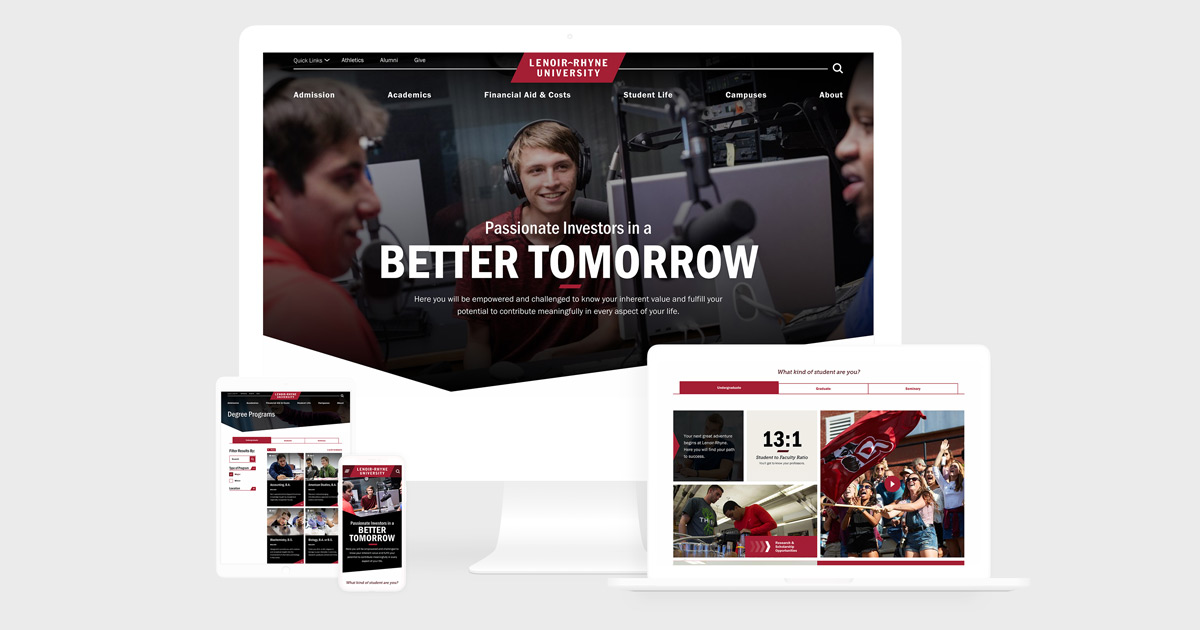This detailed caption describes a screenshot of a website template being sold, showcasing its responsive design across various devices:

"A screenshot of a website template for sale, demonstrating its responsive design on multiple devices. The main view features a computer screen displaying the full website layout, with a large header image and an indented chevron element at the bottom. Above, a black navigation bar includes five menu options: Academics, Student Life, Financial Aid, Campus, and About. In the center of the header, a red slanted tab reads ‘LeMore Ryan University.’ The heading below the image says ‘Passionate Investors: Invest in a Better Tomorrow,’ illustrated by a photo of three people engaged in a radio show, complete with microphones and headphones.

To the lower left of the computer mock-up, a mobile device screen presents a simplified, yet consistent version of the website content, with images resized and inset accordingly. To the lower right, a tablet screen depicts another variation of the template, featuring a tiled mosaic of images, emphasizing the template’s dynamic and adaptive nature. This visually appealing and versatile design resizes and adjusts seamlessly across different devices, highlighting its sophisticated programming and user-friendly interface."